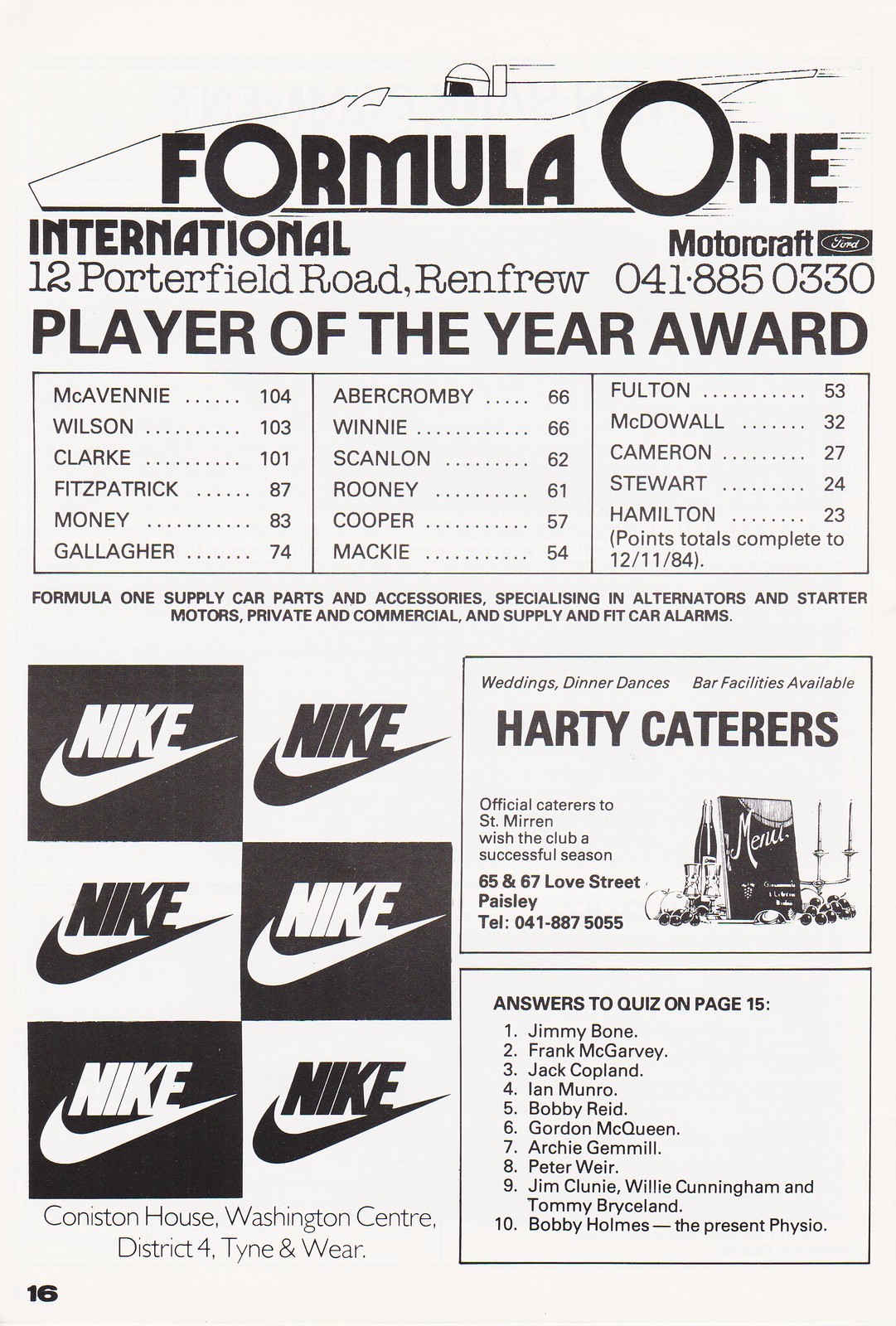This black and white pamphlet page, likely from a larger magazine dated December 11, 1984, features prominently at the top an illustrated header with stylized "Formula One" text, where the "O" letters are notably larger. Below this header, the pamphlet is titled "Player of the Year Award," displaying a three-column chart listing 18 players alongside their respective voting scores for the award: McAveney (104), Wilson (103), Clark (101), Fitzpatrick (87), Money (83), Gallagher (74), Abercrombie (66), Winnie (66), Scanlon (62), Rodney (61), Cooper (57), Mackey (54), Fulton (53), McDowell (32), Cameron (27), Stewart (24), Hamilton (23). 

The page also provides details on Formula One's specialization in car parts and accessories, located at 12 Porterfield Road, Renfrew, with the contact number 041-885-0330. Above these details is a Motocraft logo.

The lower half highlights a rudimentary Nike advertisement consisting of six alternating black and white box designs featuring the Nike logo. Adjacent to the Nike ad is a small box advertising Hardy Caterers, offering wedding and dinner dance services, and bar facilities, with contact details including a phone number and address in Paisley. The lower-left corner marks this page as page 16, while another box below the Hardy Caterers ad provides answers to a quiz found on page 15, listing names like Jimmy Bohr and Frank McGarvey. The overall presentation suggests a UK origin, possibly as part of a promotional event program or magazine from that era.